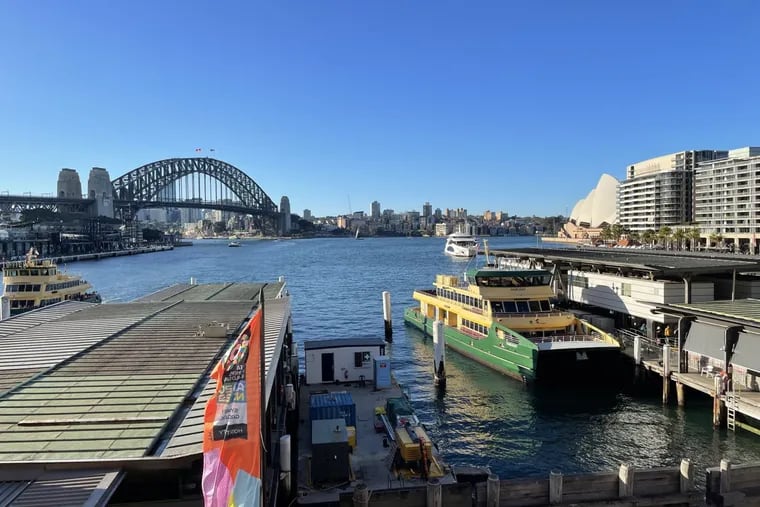The image captures a scenic view of a dock area, possibly situated in a seaport or shipyard. Dominating the left side of the frame is a short, arching bridge supported by poles rather than wires, which may function as a drawbridge. Below this, there's a boat launching platform adjacent to a rectangular structure, possibly a building or a ramp descending into the water.

On the right side, prominent features include a green and yellow tour boat docked alongside the pier. Near the boat, atop a trailer-like roof, an orange flag emblazoned with "UASIA" is visible. Another building with a flat roof, possibly a restaurant, is situated near this docked boat.

The background reveals a stunning, crystal-clear blue sky over a distant city skyline, characterized by numerous skyscrapers. An outcropping of land on the right side of the photo houses a large apartment building. In the foreground, a square asphalt area is present on the left, contrasting with the vibrant activity around the docks and water.

Overall, the image portrays a bustling waterfront scene with a variety of structures, boats, and a striking urban landscape beyond the water.